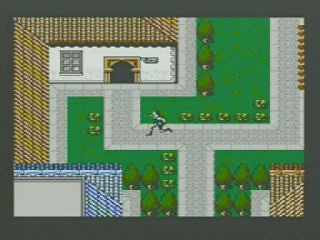In this vintage video game with pixelated graphics, the focal point is an L-shaped house situated in the top left corner, featuring a brown and tan roof, white walls, a black gaping doorway, and a gray window. A gray pathway emerges from the doorway, first extending downward to the right before continuing horizontally and then upward. In the bottom right corner is a rooftop of another building, mirroring the architectural style. Meanwhile, the bottom left corner showcases a distinct building with a blue and gray roof. The pathway is flanked by green trees on either side, enhancing the nostalgic charm of the scene. A character with skinny legs, clad in blue attire, and sporting black hair, is seen running towards the L-shaped building, adding a dynamic element to the tranquil setting.